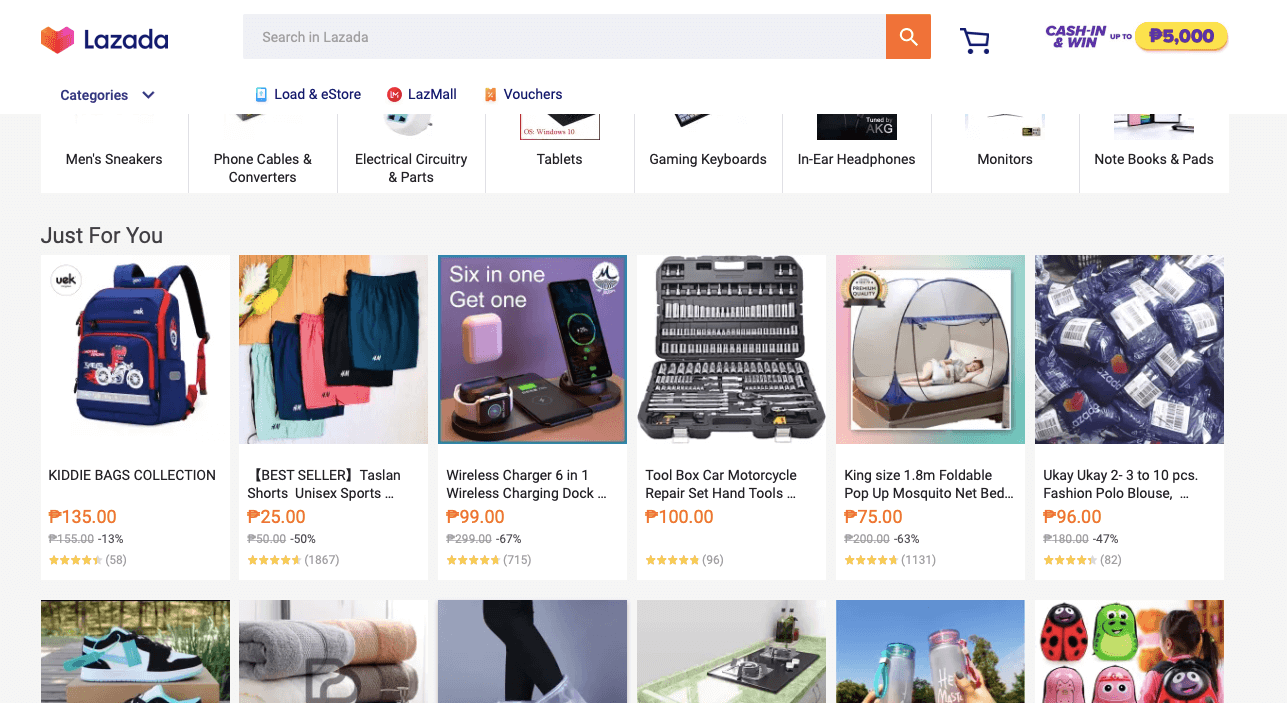The image features a clean, white background in the upper left corner. Prominently displayed in blue is the word "Lazada," spelled out as L-A-Z-A-D-A. Adjacent to it is a search bar stretching horizontally across the top of the image. To the right of the search bar, there is a blue icon depicting a shopping cart, immediately followed by text in blue that reads "Cash In and Win." Within this section, there's also a small yellow oval with blue text that reads "$5,000."

Beneath this header section, there is a menu bar listing several categories: "Categories," "Load and E-store," "LazMall," and "Vouchers." Directly under this menu, various product categories are listed in plain text: men's sneakers, phone cables and converters, electrical circuitry and parts, tablets, gaming keyboards, in-ear headphones, monitors, notebooks, and pads.

Following this, a "Just for You" section is prominently displayed, showcasing six color photos of various products. From left to right, the products include:
1. Kitty Bags Collection - Bestseller
2. Tajan Shorts - Unisex Sports
3. Wireless Charger - Six-in-One Wireless Charging Dock
4. Toolbox - Car and Motorcycle Repair Set, Hand Tools
5. King-Size 1.8M Foldable Pop-Up Mosquito Net Bed
6. UK UK 2 to 3 to 10 Piece Fashion Polo Blouse

Below this row of images, there are six more product photos, though they are partially cut off and not fully visible in the image provided.